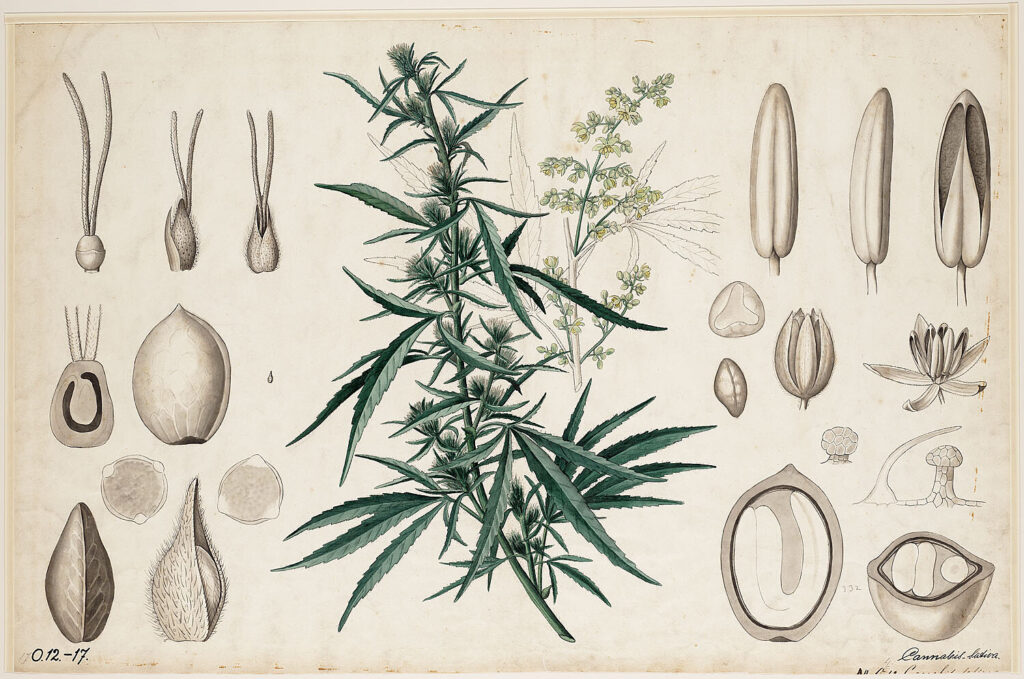The image is a detailed, artistic botanical illustration capturing various phases of a plant's life cycle. In the center, the main plant is depicted with gray-green to dark green leaves emerging from a long stem. Surrounding this main structure are softer, lighter green leaves with hints of yellow, which add depth and contrast to the composition. To the left side of the image, the life cycle is depicted starting from leaf buds at the top, progressing to budding flowers in the middle, and further down to mature leaves growing around a fruit. On the right, the illustration continues this progression, showcasing flower buds at the top, blooming flowers in the middle, and what appear to be seed pods at the bottom. The entire illustration is set against a light gray to white background. The paper appears aged, with a slightly yellowish and creased texture, suggesting an older piece of work. In the bottom right corner, there is a cursive signature, and on the bottom left, the notation "0.2-17" (or "0, 12, 17") is visible, potentially indicating the date of the artwork. This illustration resembles the structure of a day lily or a thistle and gives a comprehensive look at the various growth stages of the plant.